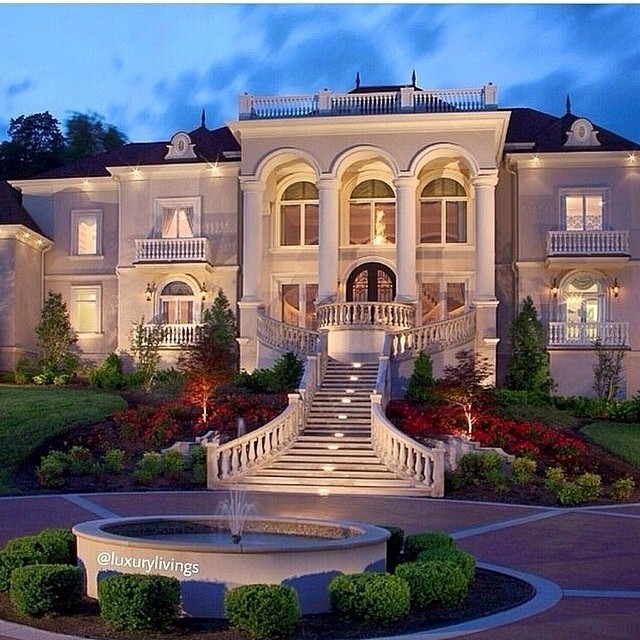The photograph showcases the front of a grand two-story manor taken slightly after dusk, with all the lights illuminating the building, against a backdrop of a dark gray sky with even darker gray clouds. Prominently featured is a round water fountain in the foreground, with several sprays of water jetting out from a central nozzle into a surrounding pool. Encircling the fountain are meticulously manicured, small square-shaped bushes set within a brown circular landscape. This area is encompassed by a paved brown roadway marked with white stripes. Leading up to the manor is an impressive grand staircase, which initially ascends as a single set of steps before splitting into two separate staircases, each branching to entrances on either side. A central black double door, elevated and framed by a decorative balcony railing, serves as the main entrance, accessible from the midpoint of the staircase where it splits. The front façade of the manor is adorned with four massive columns that support a grand overhang, beneath which lie three expansive arching windows. Additional details include lights running down the center of the staircase, enhancing the grandeur of the entryway. Small, well-maintained trees, bushes, and flowering plants decorate the base of the staircase and the perimeter of the house, adding to the lush, elegant setting. Notably, a white watermark reading "At Luxury Livings" is superimposed in the bottom left corner of the image.